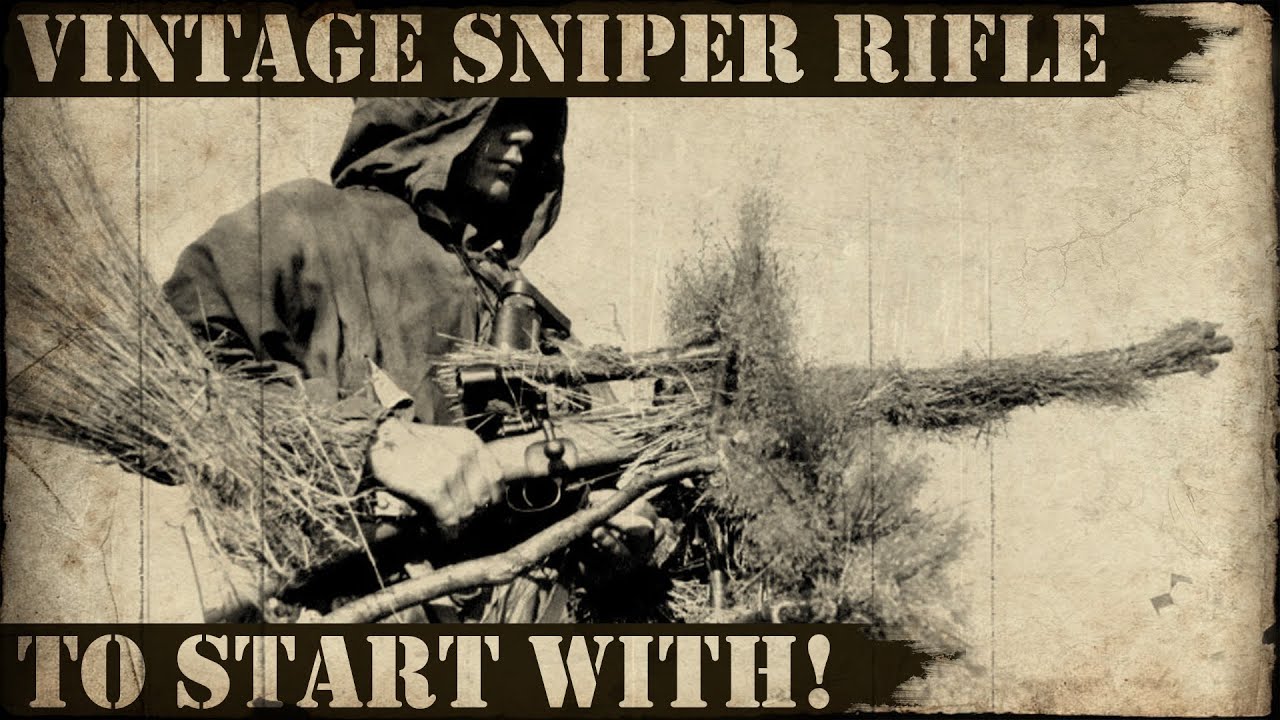This image serves as a vintage-style advertisement for a sniper rifle, conveyed through a sepia-toned font against a dark blackish-brown background. Dominating the design, the words "VINTAGE SNIPER RIFLE" are displayed prominently in all caps at the top.

Central to the composition is a person clad in a hoodie, holding a large sniper rifle that appears to be heavily camouflaged with sticks and grass, obscuring much of the gun's barrel. Despite the camouflage, the individual's right hand is visibly gripping the rifle's butt, while their left hand supports the weapon. A scope is mounted atop the rifle, though its details are hard to discern and it is not currently in use. The rifle is oriented to the right, with the rifle butt on the left side of the image.

In the bottom left corner, the phrase "TO START WITH!" is displayed in the same sepia font, adding an emphatic punctuation to the visual narrative.